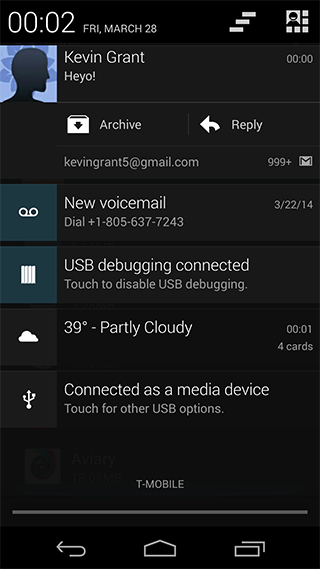The image is a screenshot set against a solid black background, capturing a display of various on-screen elements. In the upper left corner, there is a header that reads "0002, Friday, March 28th." Below this header, the name "Kevin Grant" is prominently displayed, with the time "00:00" positioned to the right of his name. Adjacent to Kevin's name, on the left, there is a generic silhouette icon representing a person. Beneath Kevin's name, there are icons for "archive" and a "reply arrow."

Directly under the "archive" icon, the text "kevingrant5@gmail.com" is shown, accompanied by "999+" indicating numerous unread emails, and the recognizable Gmail icon. Below this section, the words "new voicemail" are displayed, prompting to "dial 1-805-637-7243," with the date "3-22-14" placed to the right side.

Further down, there is a notification stating "USB debugging connected, touch to disable USB debugging." To the left of this text, there is a dark gray box containing a white square inside, which appears to be an icon related to the USB debugging notification. The image is meticulously detailed with specific timestamps, dates, icons, and actionable prompts, providing a comprehensive snapshot of the screen's content.